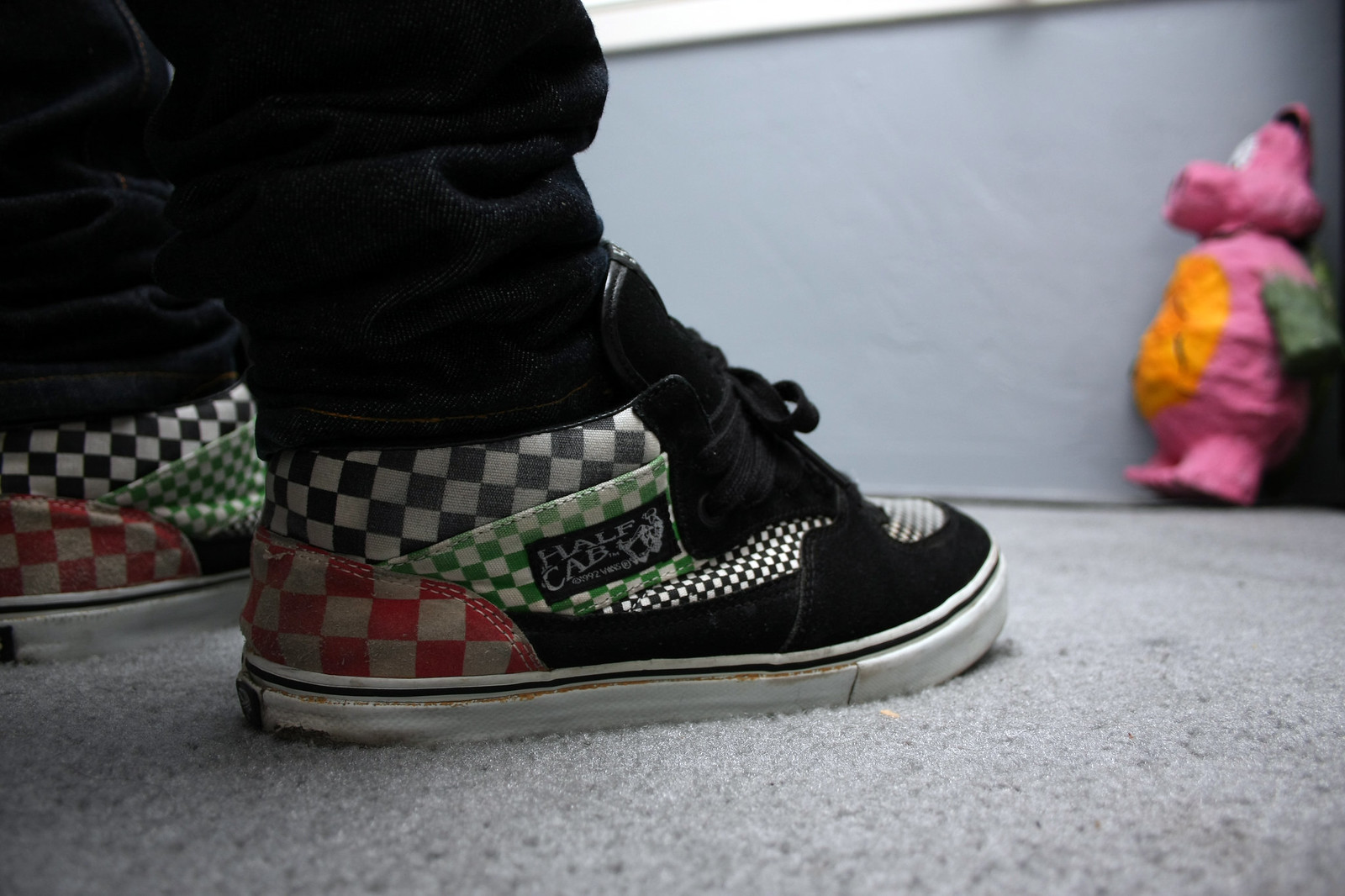This ground-level photograph captures someone’s feet adorned in vibrant high-top skateboarder shoes tagged with "Half Cab" on the side. The shoes showcase a unique checkerboard pattern: red and white checks towards the heels, green and white checks in the middle, and black and white checks at the toe and across the shoe. Accompanying the checker patterns, the shoes feature a black suede front and a white rubber rim. Despite their slightly dirty appearance, the intricate design stands out vividly. The individual, likely a child due to the shoe size, is wearing crinkled denim jeans that gather at the ankles, hinting at a longer length than necessary. They are seated or standing on a speckled grey carpet. In the background, against a possibly blue-grey wall, resides a pink papier-mâché pig or hippo toy with a yellow belly, gray marks on the arm, and large white eyes, lending a whimsical touch to the scene.